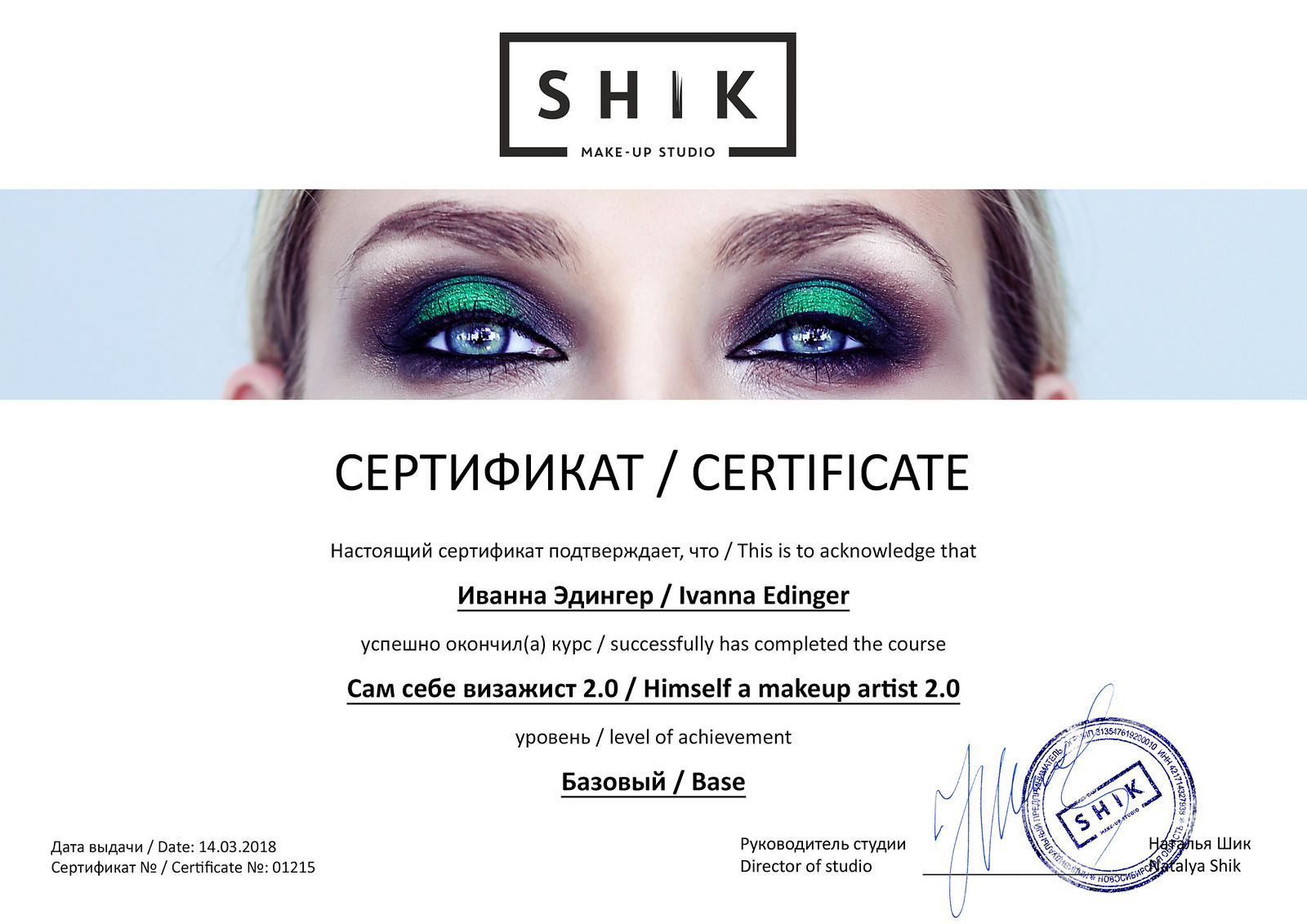The image showcases a promotional certificate with a blue background. Dominating the frame is the side profile of a woman adorned with striking makeup. She features vibrant green eyeshadow, heavily accented by dark green and purplish hues around the edges, highlighting her brown hair that frames her face on both sides.

At the top of the image, the word "Schick" appears inside a black rectangle, S-H-I-C-K, denoted in bold white letters. Beneath this, the area transitions to a solid black section, where the term "Makeup Studio" is prominent, but without a defined border.

The body of the certificate contains text in a foreign script, possibly Russian, followed by the English term "Certificate." Below this header, additional text in what appears to be Russian or Greek is present, detailing achievements. Specifically, it states "This is to acknowledge that Ivana Ettinger," followed by text in Russian which translates in part to highlight her successful completion of a course.

Further, it mentions that Ivana Ettinger has achieved the status of "Makeup Artist 2.0," praised in both Russian and English. The document concludes with more text in the foreign script, acknowledging the "Level of Achievement" and indicating "Base" as the level. A distinctive stamp is also present, affirming the authenticity of the certificate, reinforcing the idea that the text is predominantly in Russian or a similar language.